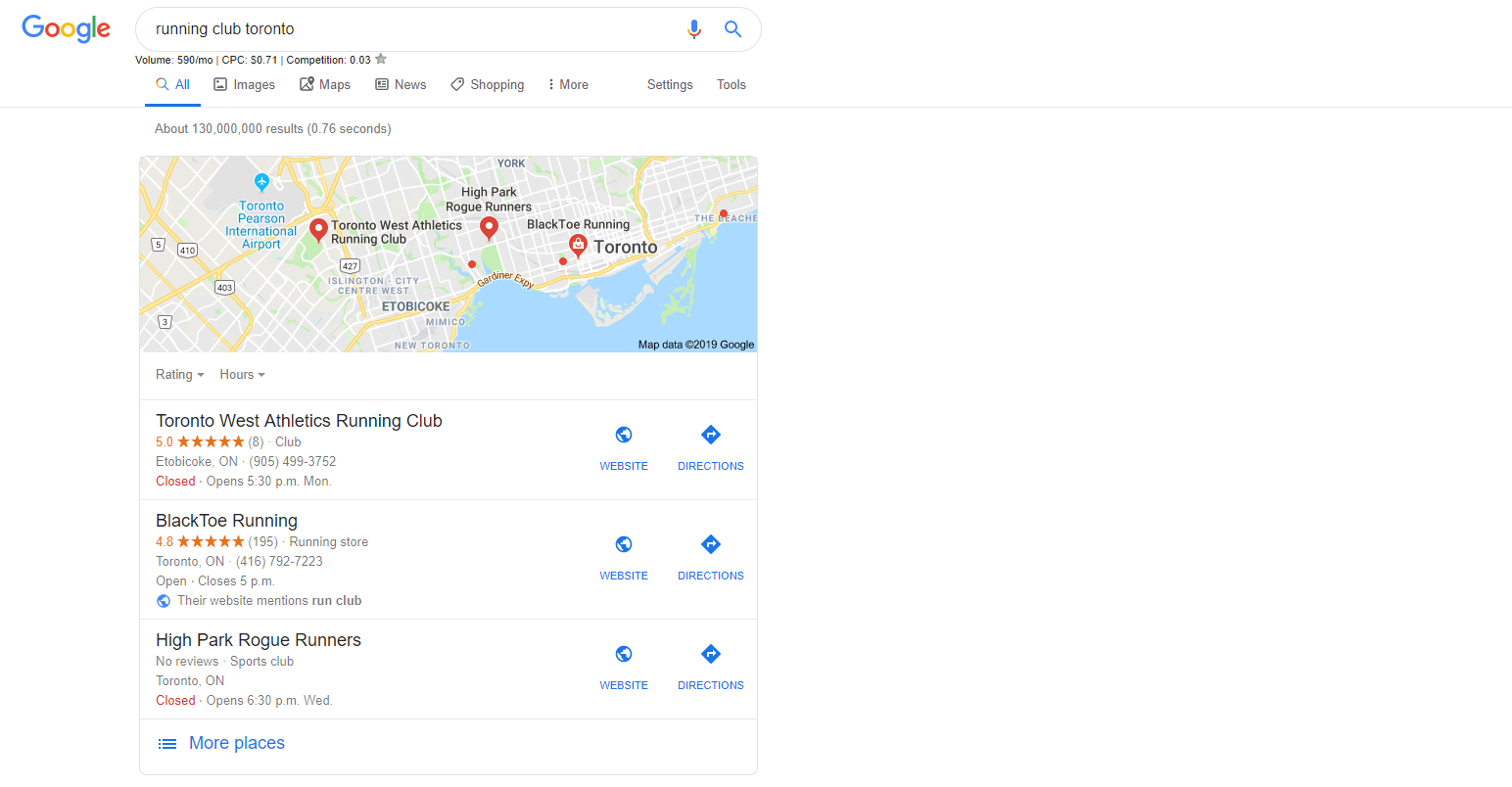The image captures a Google search results page for the query "Running Club Toronto." At the top left of the image, the iconic Google logo is prominently displayed with its distinct color scheme: a blue 'G', a red 'O', a yellow second 'O', a blue second 'G', a green 'L', and a red 'E'. Adjacent to the logo is the elongated horizontal search bar, within which "Running Club Toronto" is typed in black text. To the top right of this search bar, there are two icons: a grey microphone symbol for voice search and a grey magnifying glass symbol to initiate the search.

The primary navigation menu below the search bar and logo includes tabs labeled "All," "Images," "Maps," "News," "Shopping," "More," "Settings," and "Tools." The central part of the image showcases a Google Maps snippet highlighting various running clubs in Toronto. Notable labels on the map include "Toronto," "Black Toe Running," "High Park Road Runners," and "Toronto West Athletics Running Club."

Beneath the map, three detailed sections offer more information about specific running clubs. The first section is for "Toronto West Athletics Running Club," boasting a five-star rating. The second section highlights "Black Toe Running," which has a 4.8-star rating. The third section features "High Park Road Runners," which has yet to receive any reviews.